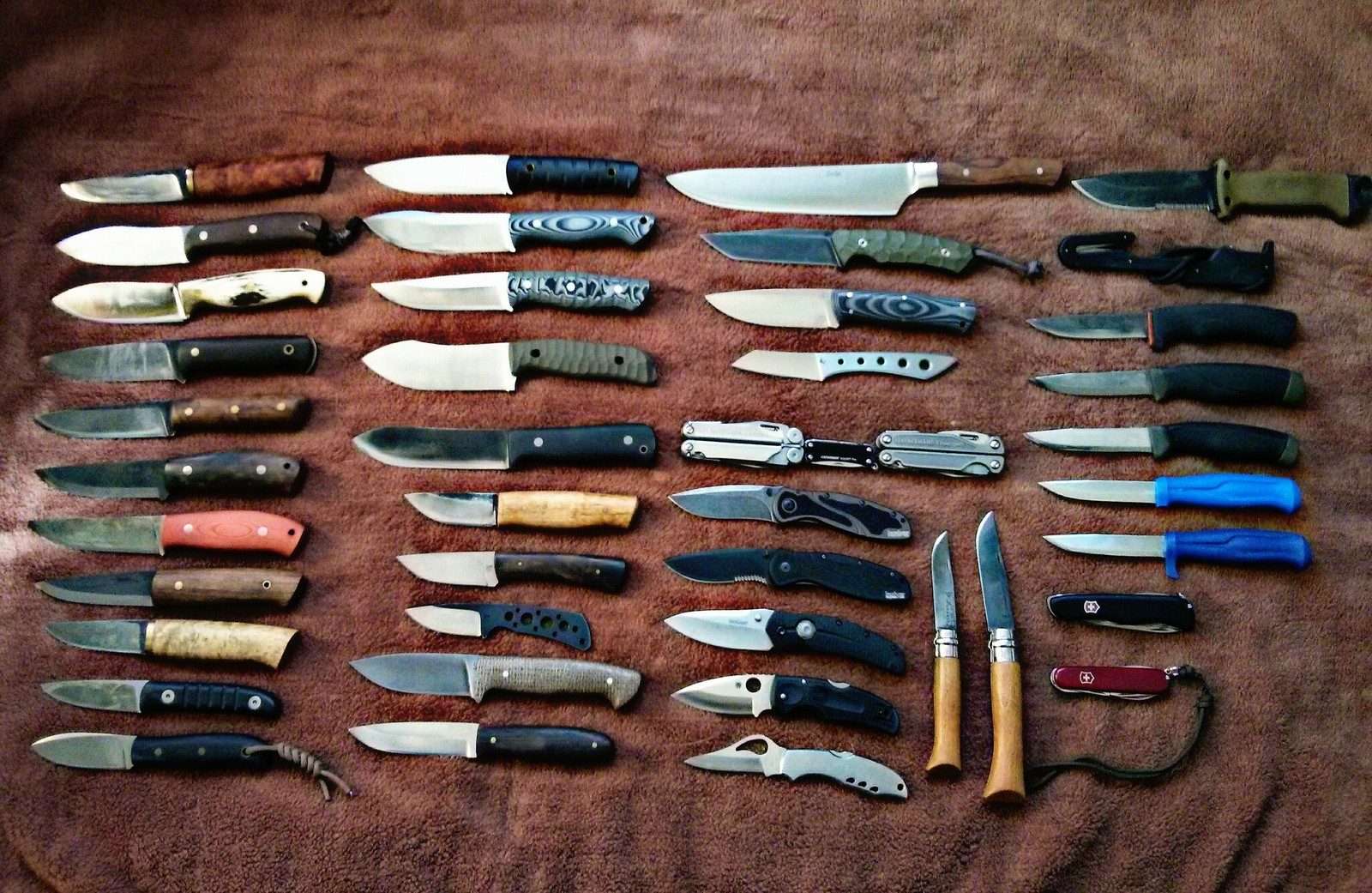The photograph showcases an extensive knife collection, meticulously laid out on a reddish-purple, plush blanket or towel. There are approximately 30-40 knives in total, each positioned with the blades facing left and the handles oriented to the right, creating a neat, parallel arrangement. Exceptions include two pocket knives in the lower right corner, which remain closed, and a few upright knives adjacent to them. The collection features a diverse array of knife types and handle designs, with a spectrum of colors including black, blue, brown, grey, green, and a unique pinkish hue. Handle materials vary from wood to plastic, with some knives sporting camouflage patterns or simple solid colors. Most of the knives are fixed-blade, although there may be a butterfly knife among them. The display reveals signs of use and frequent sharpening, indicating they are well-maintained.